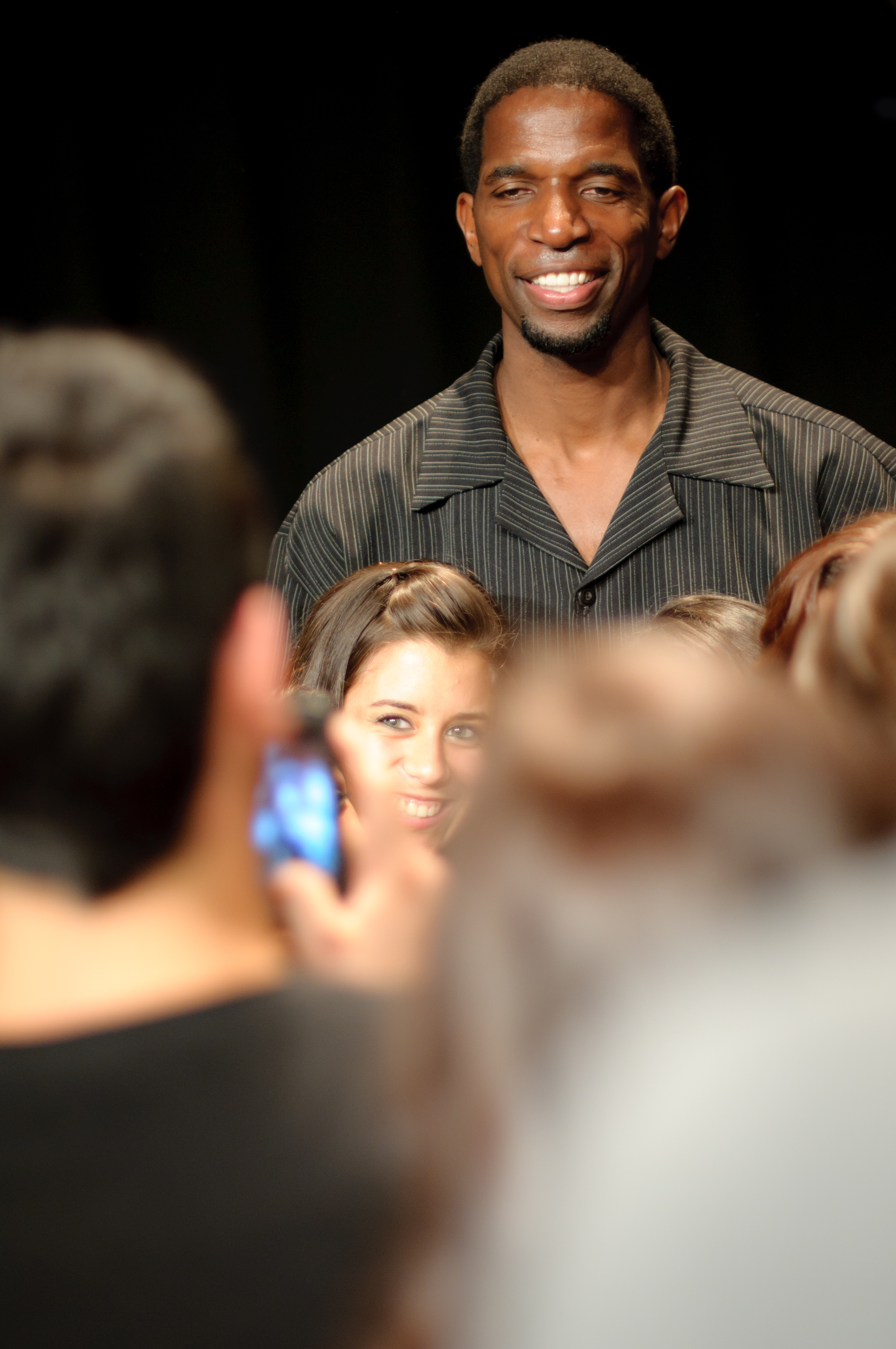A tall African-American man with short black hair stands against a black background, smiling broadly at the camera. He wears a distinctive black and white striped shirt that appears silk-like. In front of him stands a Caucasian woman with long brown hair and vibrant blue eyes, also smiling warmly. To their left, a man with short black hair in a black t-shirt holds a phone, capturing the moment. To the right, a blurred figure in a gray shirt faces the couple, possibly also taking a photo. Another person with short auburn hair can be seen near the edge of the frame. The scene captures a joyful moment, with onlookers and background elements intentionally blurred to focus on the central, smiling figures.